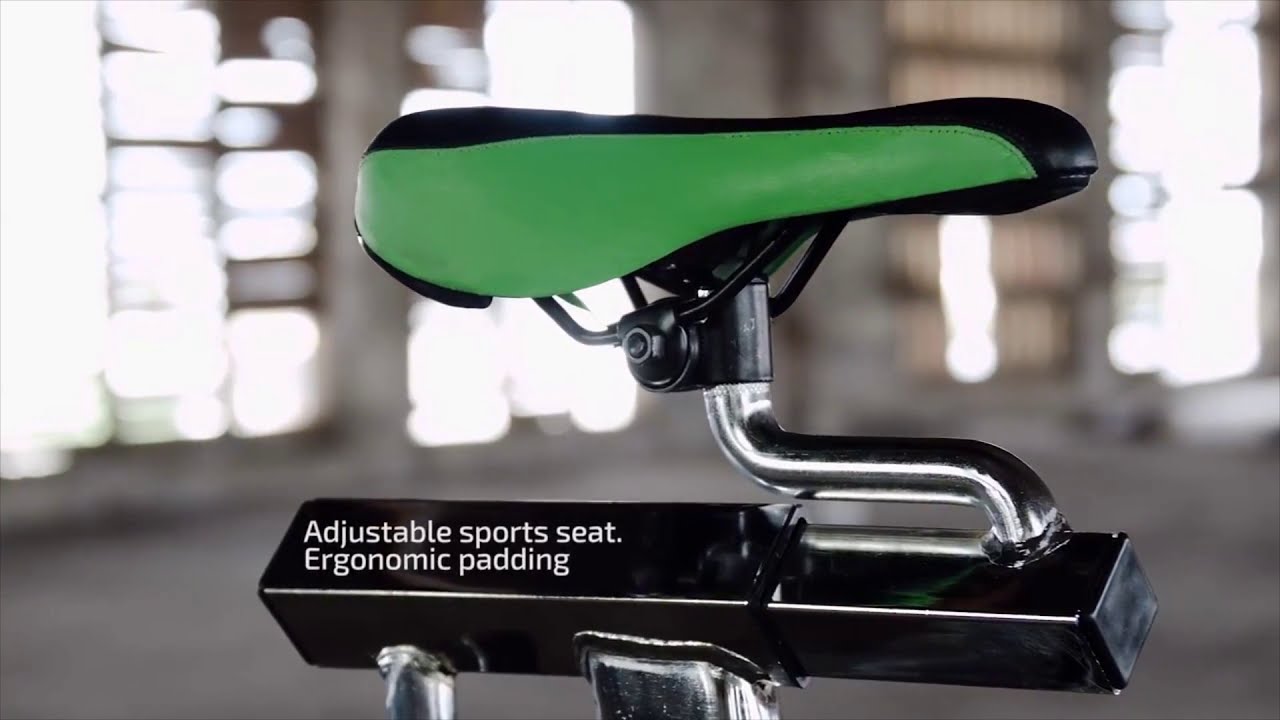The image features a close-up view of a bicycle seat designed for advertisement purposes. The bike seat boasts a sleek design with its main part upholstered in black leather, complemented by lime green leather trim on the sides. It is connected to a silver metal bar, which extends into a black metal support rod. Inscribed on this black rod are the words: "adjustable sports seat, ergonomic padding," indicating its adjustable nature and focus on comfort. The background is notably blurred, featuring indistinct lights and gray cement walls, which draws all focus to the seat itself. The overall appearance is premium and intended to entice prospective buyers with its modern and ergonomic design.